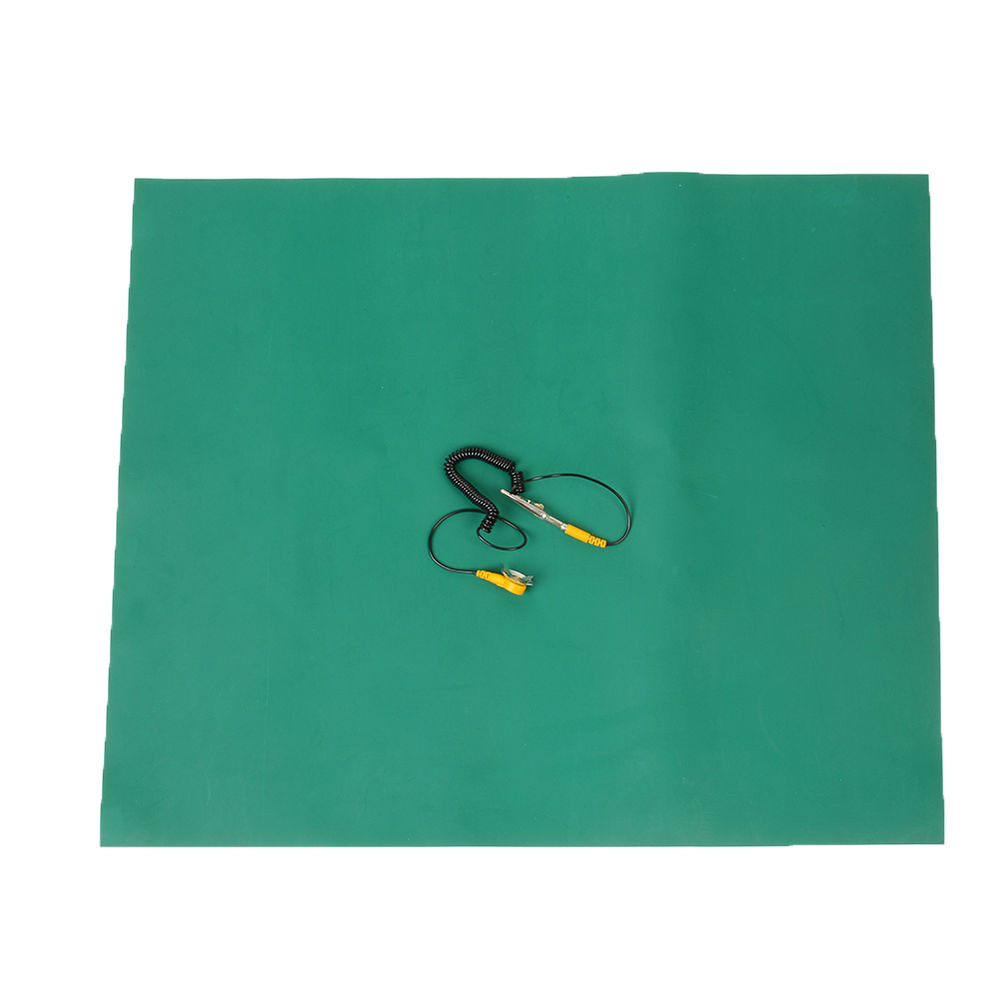This photograph features an unidentified electronic cable resting on a dark green, slightly uneven surface, possibly a piece of paper with a crease towards the right-hand side. The central element of the image is a tightly wound black plastic coil, reminiscent of a telephone cord, measuring approximately four to six inches. Emerging from each end of this coiled section are two thinner black wires, each extending a few inches. On the left end, the wire is terminated with a yellow covering and a metallic alligator clip, seemingly designed as a strain relief. The opposite end of the wire concludes with another yellow strain relief, attached to a small, spiked metal disc. The entire setup suggests a utilitarian design possibly related to electronics or laboratory use, although the specific function remains unclear. The vivid green background contrasts with the cable, drawing focus to the central object.